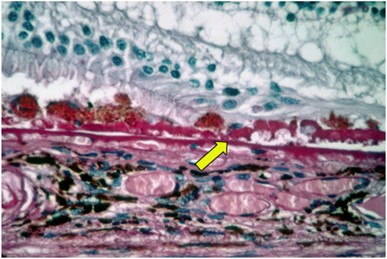This image resembles a page from a medical textbook, depicting a detailed, stained cross-section of skin tissue viewed under a microscope. The background is predominantly white, with the top portion featuring white and green hues and small brown and green circles. Below this, there's a thin layer of brown and red pigments. The central part of the image showcases a bright pinkish-purple horizontal barrier, possibly indicating the epidermal layer, with a prominent yellow arrow pointing directly at it. Underneath this barrier, the tissue is stained in pink and red shades, interspersed with aqua and black ovals, giving it an appearance akin to raw meat. The lower half consists of more flattened cell structures, continuing the pink and red coloration mixed with similar green and black as seen at the top. Overall, this image highlights the stratified layers of the tissue, emphasizing the demarcation indicated by the arrow, and bears the meticulous detailing characteristic of educational materials.